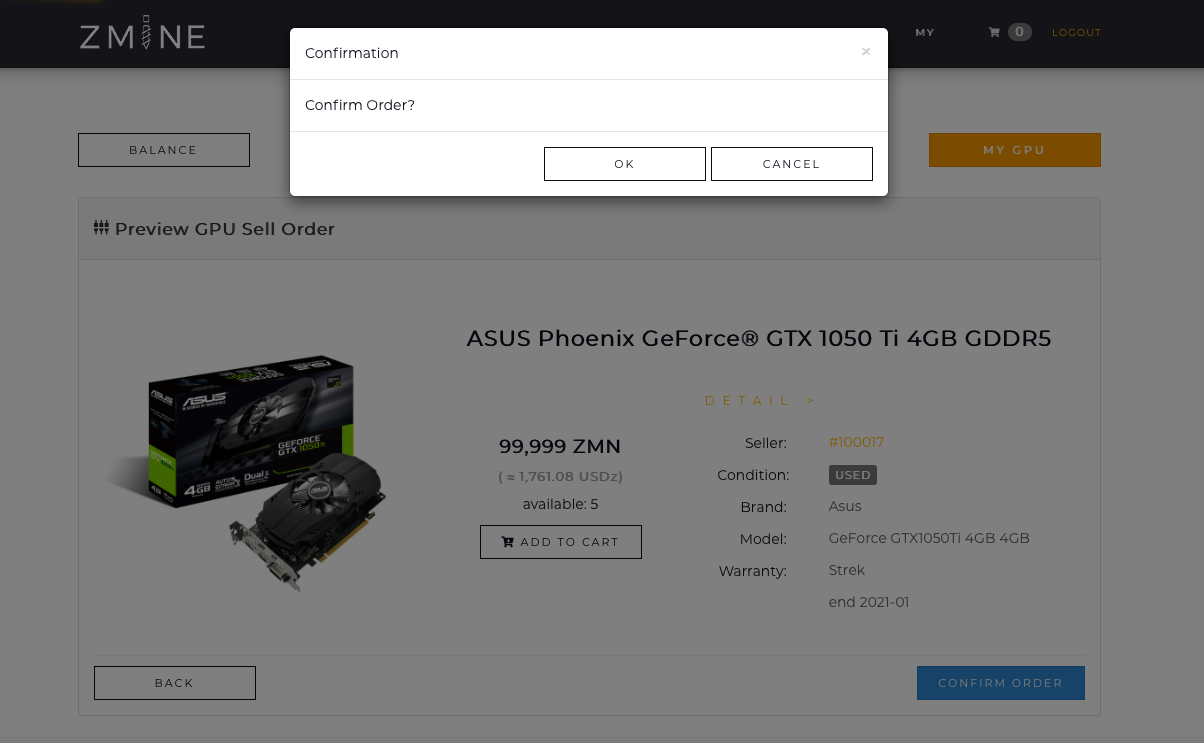In this horizontal rectangular screenshot, the focal point is a small highlighted rectangular box located at the upper center of the image. The box consists of gray text displaying "Confirmation" and "Confirm Order," with two options below: "Okay" and "Cancel."

The background reveals a web page, presumably from the website "ZMINE." On the lower left side of the page, beneath the site name, there is a section labeled "Balance." Below this, we see a highlighted box containing a preview of a GPU sales order. The details within the box are as follows:

- Item: "Asus Fenix GeForce GTX 1050 Ti 4GB GDDR5"
- Price: "99,999 ZMN"
- Available: "5 units"
- Option to: "Add to Cart"
- Seller ID: "100017"
- Condition: "Used"
- Brand: "Asus"
- Model: "GeForce GTX 1050 Ti 4GB GDDR5"

This well-detailed screenshot effectively highlights a user nearing the completion of an order on the ZMINE platform.